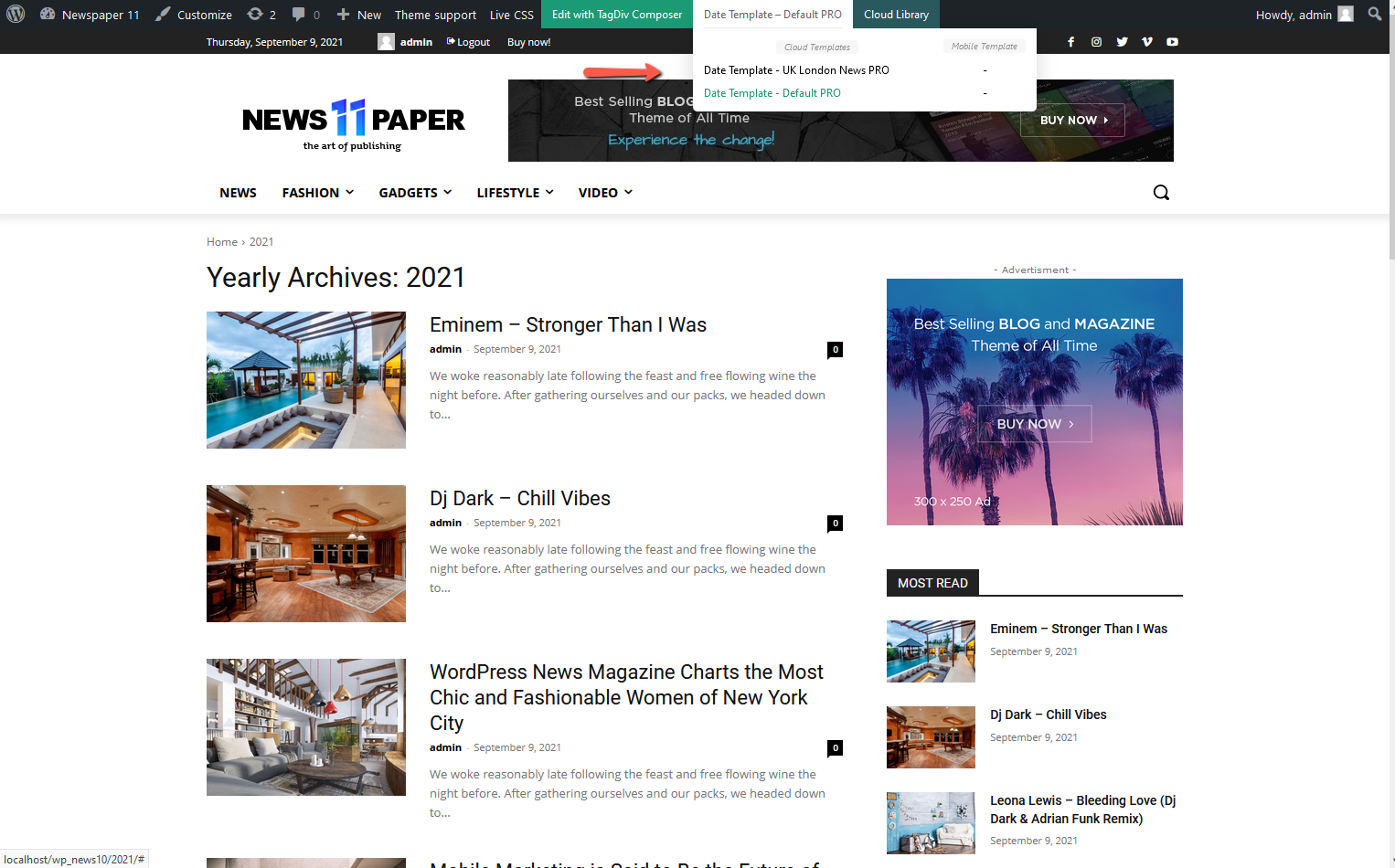This description provides an overview of a web page from the "News 11 Paper" website, with a focus on its WordPress-driven interface and content layout:

---

Displayed is a sleek and modern webpage from the "News 11 Paper" website, with "11" stylishly embedded within the name. The header boasts a solid black background typical of a WordPress template. Key elements in the top board include:

- A tab for customization options.
- A chat feature.
- An addition symbol for adding new elements.
- A tab labeled "Theme Support."
- A "Live CSS" option for real-time styling adjustments.

A prominently visible green tab labeled "Edit with Tagline Composer" stands out, accompanied by a dropdown menu with a red arrow pointing to it. This menu offers several date templates such as "Default PRD," "UK London News Pro," and "Default Pro" for advanced editing features.

Additionally, the interface includes a "Cloud Library" option and a set of social media icons or logos including Facebook, Instagram, X (formerly known as Twitter), Vine, and YouTube. A personalized greeting, "Howdy Admin," appears next to a space for a user photo and a search button. Below this, various navigation tabs are available for categories like:
- News
- Fashion (with a dropdown arrow)
- Gadgets (with a dropdown arrow)
- Lifestyle (with a dropdown arrow)
- Video (with a dropdown arrow)

The main content section features a 2021 archive labeled "A Home". The visual highlight is a lavish home showcasing an inviting pool adjacent to its deck, followed by the title "Eminem - Stronger Than I Was." Further down, a sumptuous living area is depicted, headlined by "DJ Stark - Chill Vibes." Another luxurious home image accompanies titles highlighting high-end properties, including "WordPress New Magazine Charts: The Most Chic and Fashionable Women of New York City."

To the right, an advertisement promotes the "Best-Selling Blog and Magazine Theme of All Time," inviting purchases. The "Most Read" section summarizes popular content:
- Eminem - Stronger Than I Was
- DJ Stark - Chill Vibes
- Leona Lewis - Bleeding Love (Dark and Adrian Funk Remix).

---

This detailed caption encapsulates the interactive elements, content, and overall structure of the webpage, providing a comprehensive overview for viewers.